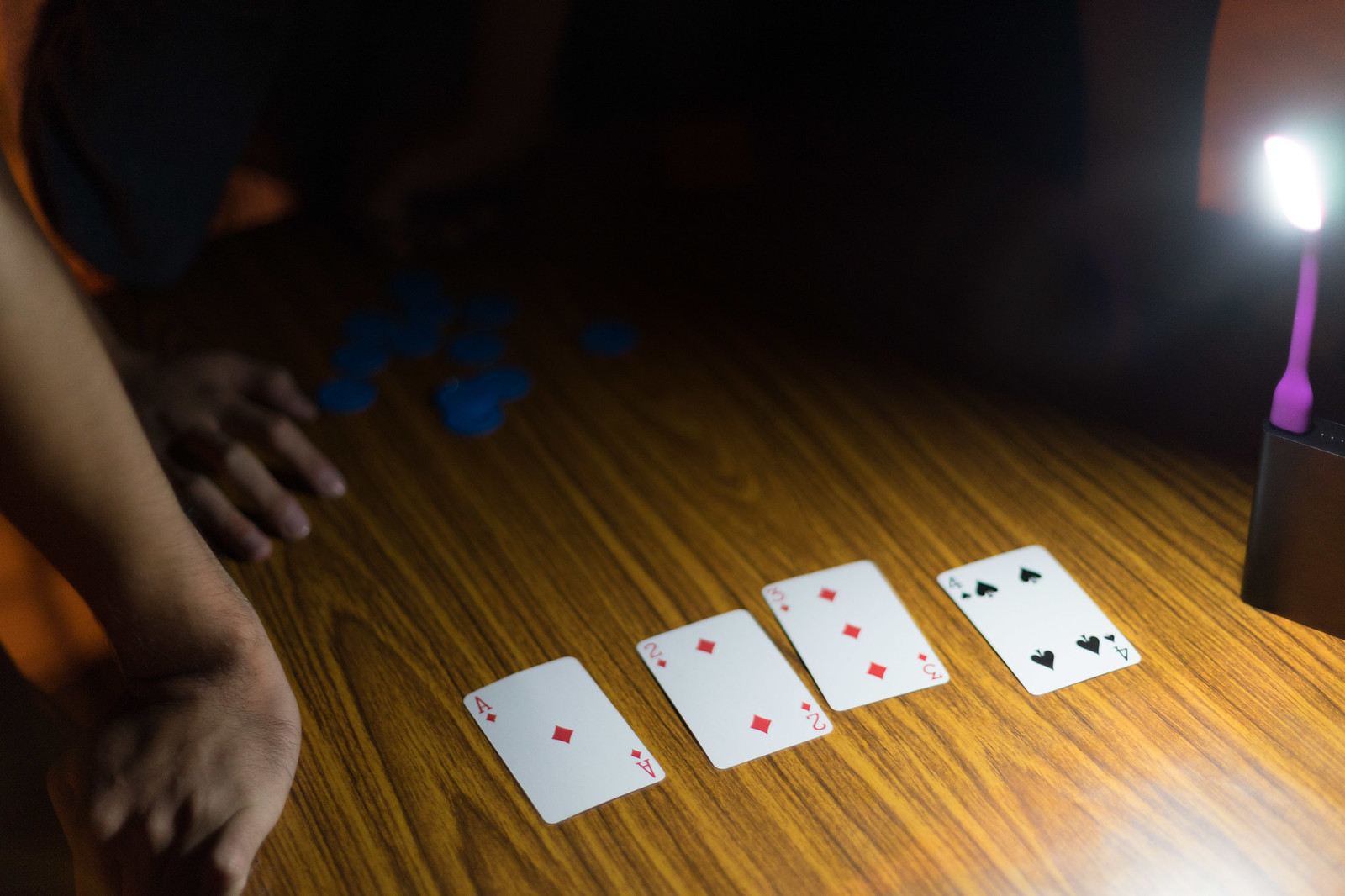In a dimly lit setting with a dark background, a brown table is situated at the forefront. Toward the back of the table, a stack of blue poker chips is visible. On the table, there are two distinct hands, belonging to different individuals, both resting beside four playing cards. The cards displayed are the four of spades, three of diamonds, two of diamonds, and the ace of diamonds. On the edge of the table, there is a small black plastic square emitting a bright purple light, illuminating the cards distinctly. Additionally, a red fabric, either a towel or a curtain, hangs behind the light, contrasting against the dark surroundings. The scene is stark, with the focus primarily on the illuminated cards and the subtle details within the low-lit environment.